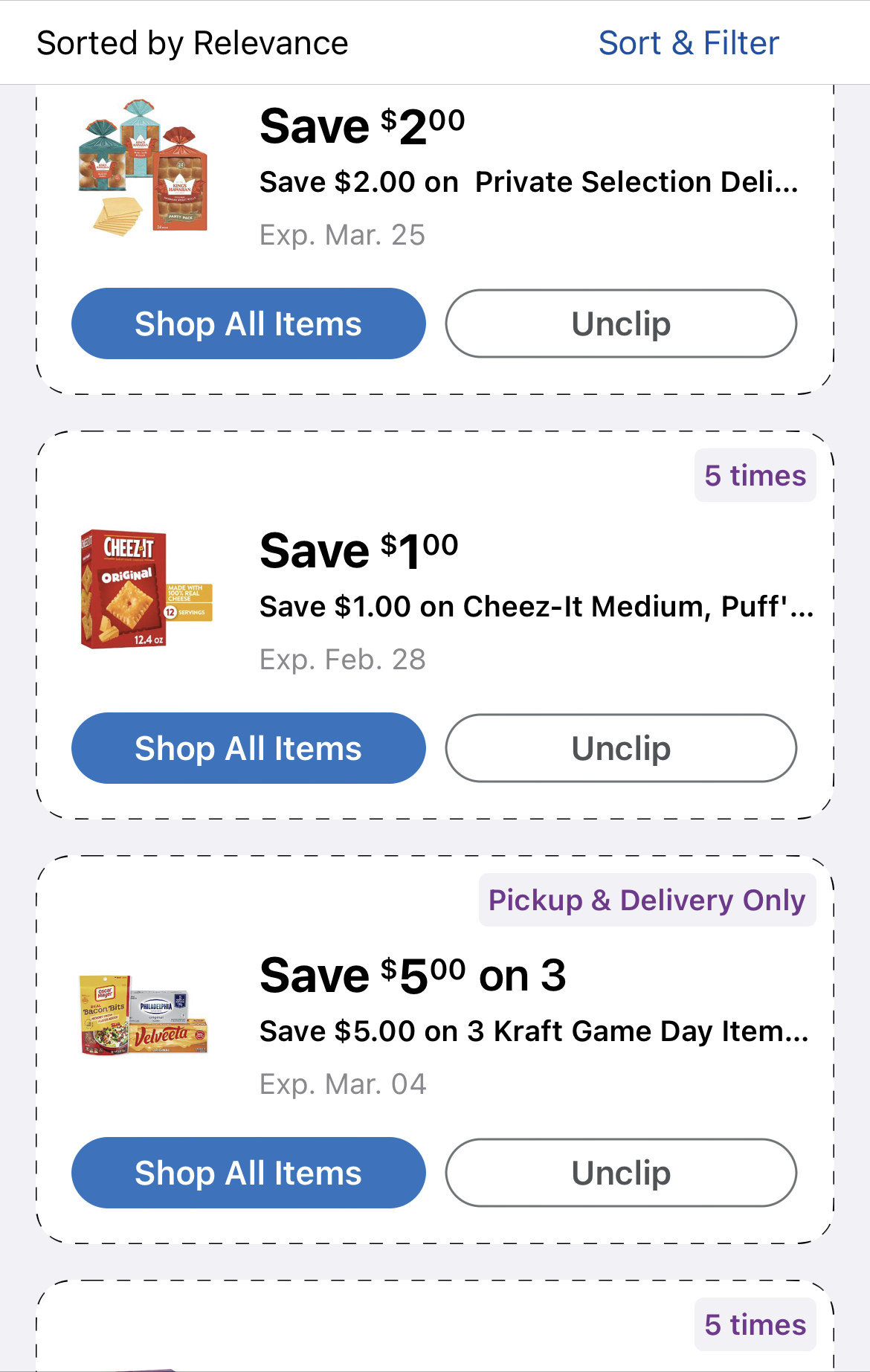This image is a screenshot captured from a smartphone in portrait mode, displaying a grocery shopping app's coupon section. The background is predominantly white or light gray. At the top, the interface indicates that the items are "Sorted by relevance." In the upper right corner, there is an option labeled "Sort and Filter" in blue text.

The first section displays a coupon with a text header "Save $2 on Private Selection Deli," which expires on March 25th. There are options for "Shop All Items" or "Unclip." On the left side, there is an image representing the Private Selection Deli.

The next section offers a coupon for "Save $1 on Cheez-It Medium," expiring on February 28th, along with the "Shop All Items" button in blue.

Following that, there is a row marked "Pickup and Delivery Only," featuring a coupon to "Save $5 on three Kraft Game Day items." There is a note that this offer is "5x," indicating the coupon can be used up to five times. The associated button also allows users to "Shop All Items."

Each of these sections includes a blue "Unclip" button, signifying that these coupons have already been clipped by the user. The inclusion of terms like "Pickup and Delivery Only" implies certain restrictions on how these coupons can be redeemed.

Overall, this screenshot provides a detailed view of multiple digital coupons available for use within a grocery shopping app, highlighting the functionality, expiration dates, and specifics of each offer.